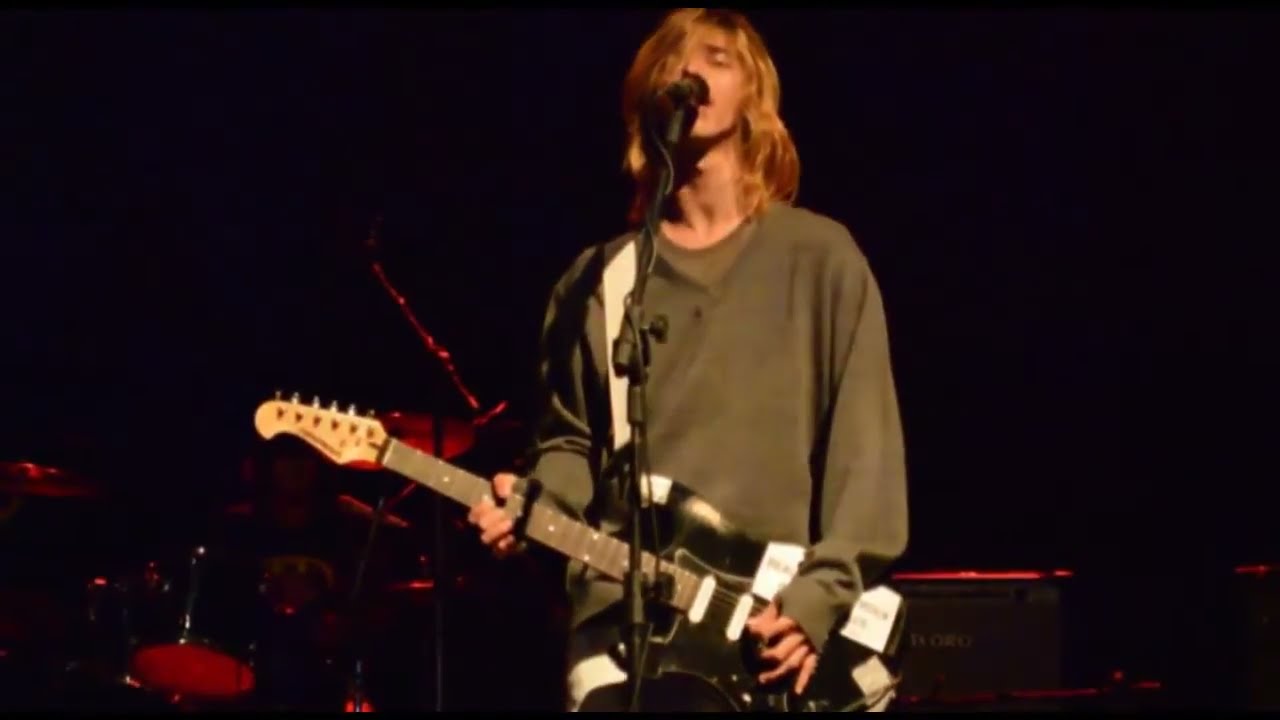This horizontal rectangular image depicts a musician who closely resembles Kurt Cobain from the band Nirvana, performing on stage. He is captured in the act of singing into a microphone, with the mic positioned right up to his mouth, suggesting intense engagement with his performance. He sports a loose-fitting, baggy dark green sweater, possibly layered over a grayish top, and has long, mildly messy blond hair. Both his hands are occupied with a black guitar, strumming with one hand while the other sets the notes. The performer's eyes are somewhat closed, adding to the sense of immersion in his music.

The background is predominantly dark, with faint visibility of instruments and speakers that are subtly illuminated by a reddish tint. There is a splash of red on the left side, possibly a chair, and a door with red light seeping from underneath, contributing to the overall intimate and somewhat mysterious ambiance of the setting.